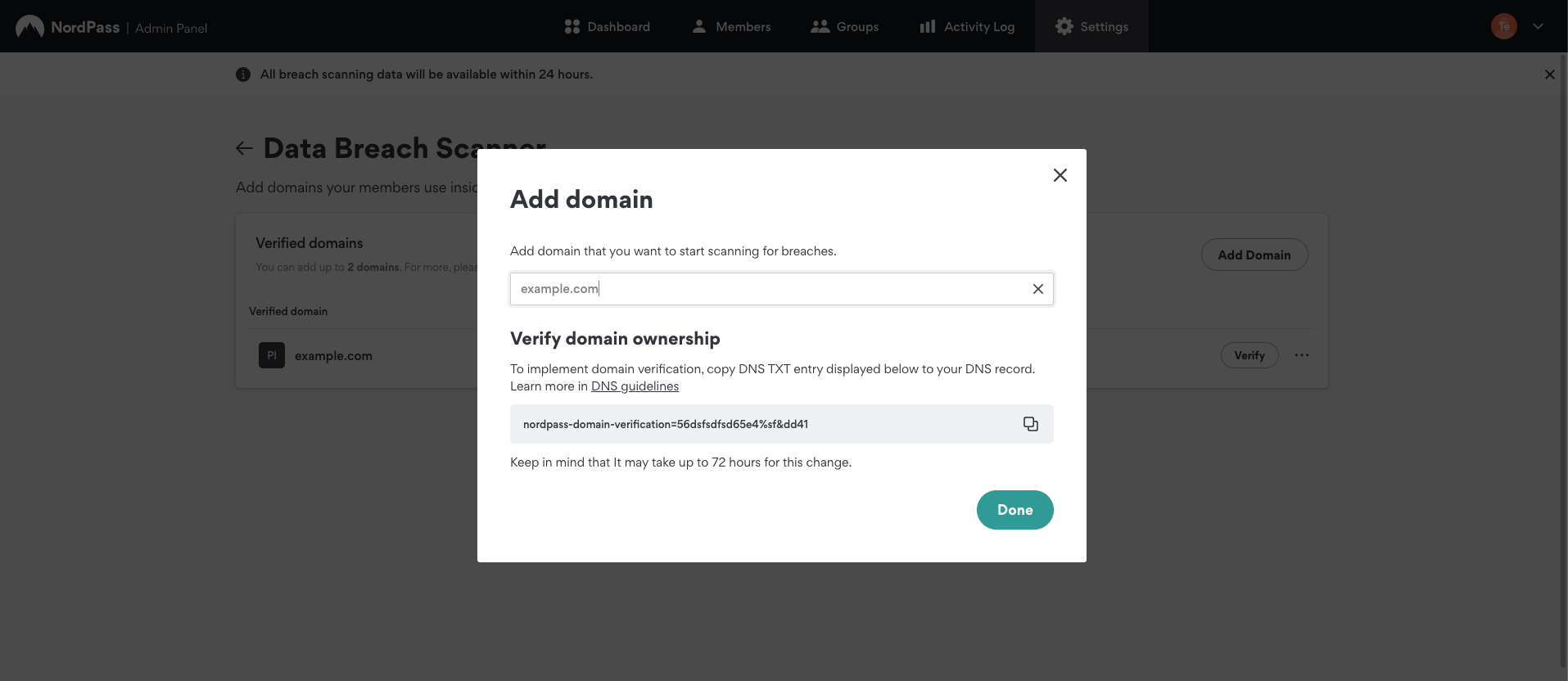The screenshot showcases a web page from the NordPass website, prominently featuring an "Admin Panel" interface. The top banner is black, adorned with the NordPass logo on the upper left—a white circle with an unspecified icon inside—accompanied by the text "NordPass Admin Panel." The central focus of the page is a white, interactive box where users need to enter information.

Within the black top banner, several navigation options are visible:
- "Dashboard," symbolized by four square icons.
- "Members," denoted by a single silhouette icon.
- "Groups," illustrated with two silhouette icons.
- "Activity Log," indicated by three horizontal bars.
- "Settings," represented by a gear icon.
On the far right of the banner, an orange circle likely identifies the user, accompanied by a downward pointing arrow for additional options.

Below this banner, the background transitions to white. A gray circle with an eye icon contains the text: "All breach scanning data will be available within 24 hours." Adjacent to this, the text "Data Breach Scanner" appears, though partially obscured by the central white box.

Within the central white box, the header "Add Domain" appears at the upper left, while a close "X" button resides at the upper right. The instructions below the header read, "Add domain that you want to start scanning for breaches," followed by an input box pre-filled with "example.com." Next to the input box is an "X" icon for removal.

Further instructions provide a step to "Verify domain ownership," directing users to "copy the DNS TXT entry displayed" (with the remaining text unclear) into their DNS record for verification. A gray bar underneath contains further unspecified instructions. 

In the far right of this bar, a gray icon resembling multiple windows is present. Below, another message warns, "Keep in mind that it may take up to 72 hours for this change."

In the bottom right corner of the white box, a green "Done" button with white text allows users to finalize their entries.